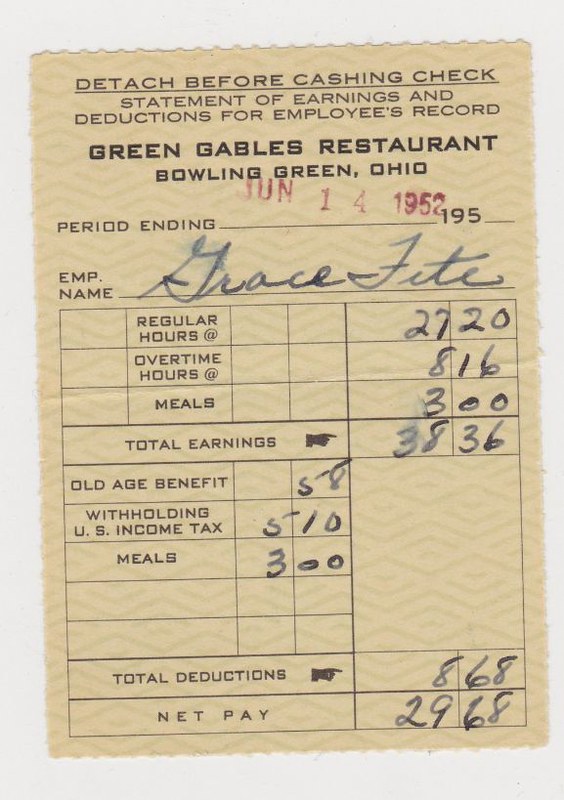The image displays an old pay slip from 1952, centered on and flat against a solid white or gray surface. The pay slip, primarily beige with ink and pencil details, has a pattern of tiling diamonds in the background. The top of the slip is inscribed with "Detach Before Cashing Check, Statement of Earnings and Deductions for Employee's Record," followed by "Green Gables Restaurant, Bowling Green, Ohio." A date stamp in red ink, "June 14, 1952," appears just below. The pay slip details the earnings of Grace Fite, an employee who worked 27.2 hours with an additional 8 hours and 16 minutes of overtime, earning $38.36 for the period, likely a week. There are deductions for U.S. income tax ($5.10), meals ($3.00), and old age benefit ($58), which sum up to a total deduction of $8.68, leading to a net pay of $29.68. The image is devoid of any notable background, making the pay slip the sole focal point.